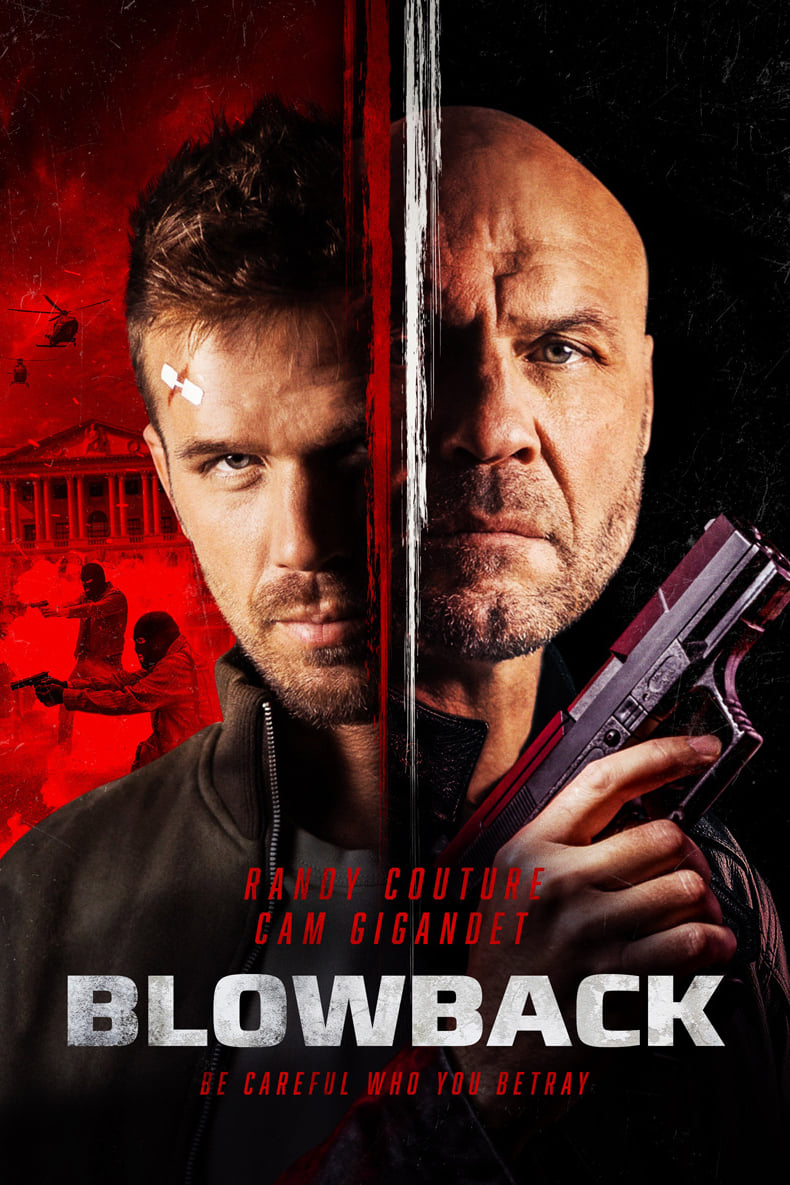The movie poster prominently features the juxtaposed faces of two men, split down the middle by a jagged, painted-looking line. On the left side is a slightly younger man with brown hair, dark eyes, a mustache, and a beard, set against an apocalyptic red and black background. This backdrop includes masked men with guns appearing ready to shoot, a building, and a helicopter in the sky. On the right side is an older, bald man with a beard and mustache, holding a pistol near his face, with a stark black background behind him. Both men are scowling, adding to the intense, brooding atmosphere. The poster prominently displays the names "Randy Couture" and "Cam Gigandet" in red, with the movie title "Blowback" in large white capital letters, followed by the tagline "Be Careful Who You Betray" in smaller red capital letters. The vivid contrast between the red, chaotic background and the black, empty space underscores the movie's themes of betrayal and conflict.